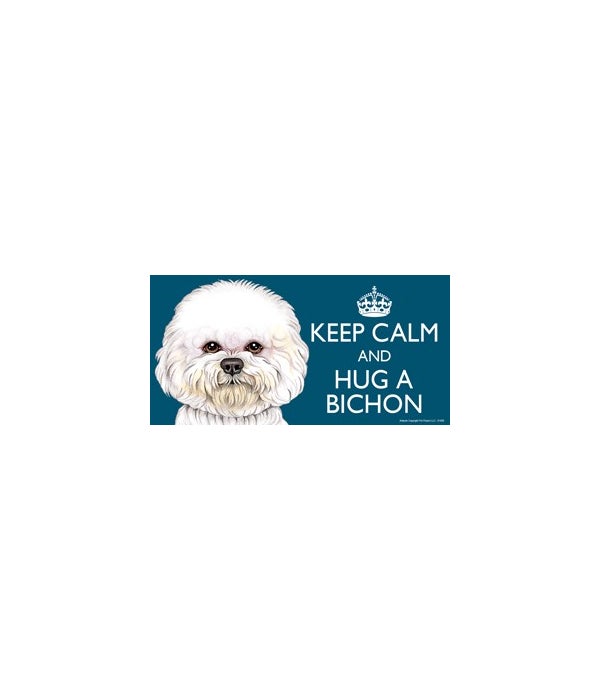The image is a small, horizontally aligned rectangular banner with a dark turquoise blue background. On the left side is a detailed drawing of a Bichon Poodle with white, fluffy fur that has hints of tan and gray in certain areas. The dog features shiny, black beady eyes and a somewhat shiny blackish-gray nose; its mouth is not very visible. The right half of the image displays a classic World War II-era "Keep Calm" message with a white stylized crown at the top, followed by the text: "KEEP CALM AND HUG A BICHON.” All the text is in capitalized, sans-serif font and white in color, maintaining the traditional style of the iconic British slogan.